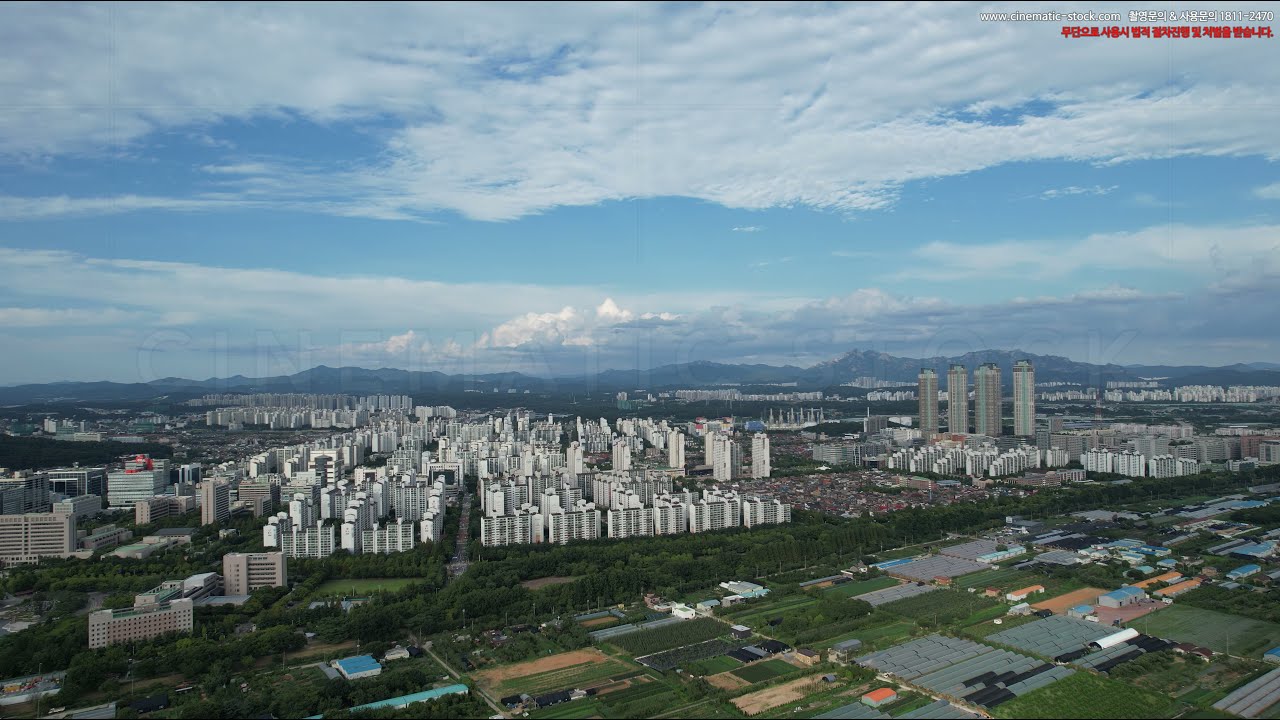The photograph captures an expansive cityscape under a partly cloudy, blue sky, showcasing a variety of cloud formations with thicker clouds framed against a mountainous or hilly horizon. The central portion of the image features a dense array of tall, uniform buildings, including several skyscrapers and numerous large apartment complexes that dominate the downtown area. The foreground presents a contrast with flat, sectioned fields, possibly agricultural land, interspersed with lines of trees and crisscrossing roads. Further down, a more residential zone is visible, characterized by smaller streets, grassy areas, and clusters of trees. A small, difficult-to-read row of white and red print is noted in the upper right-hand corner, but the primary focus remains on the vibrant juxtaposition of urban density and natural landscapes.